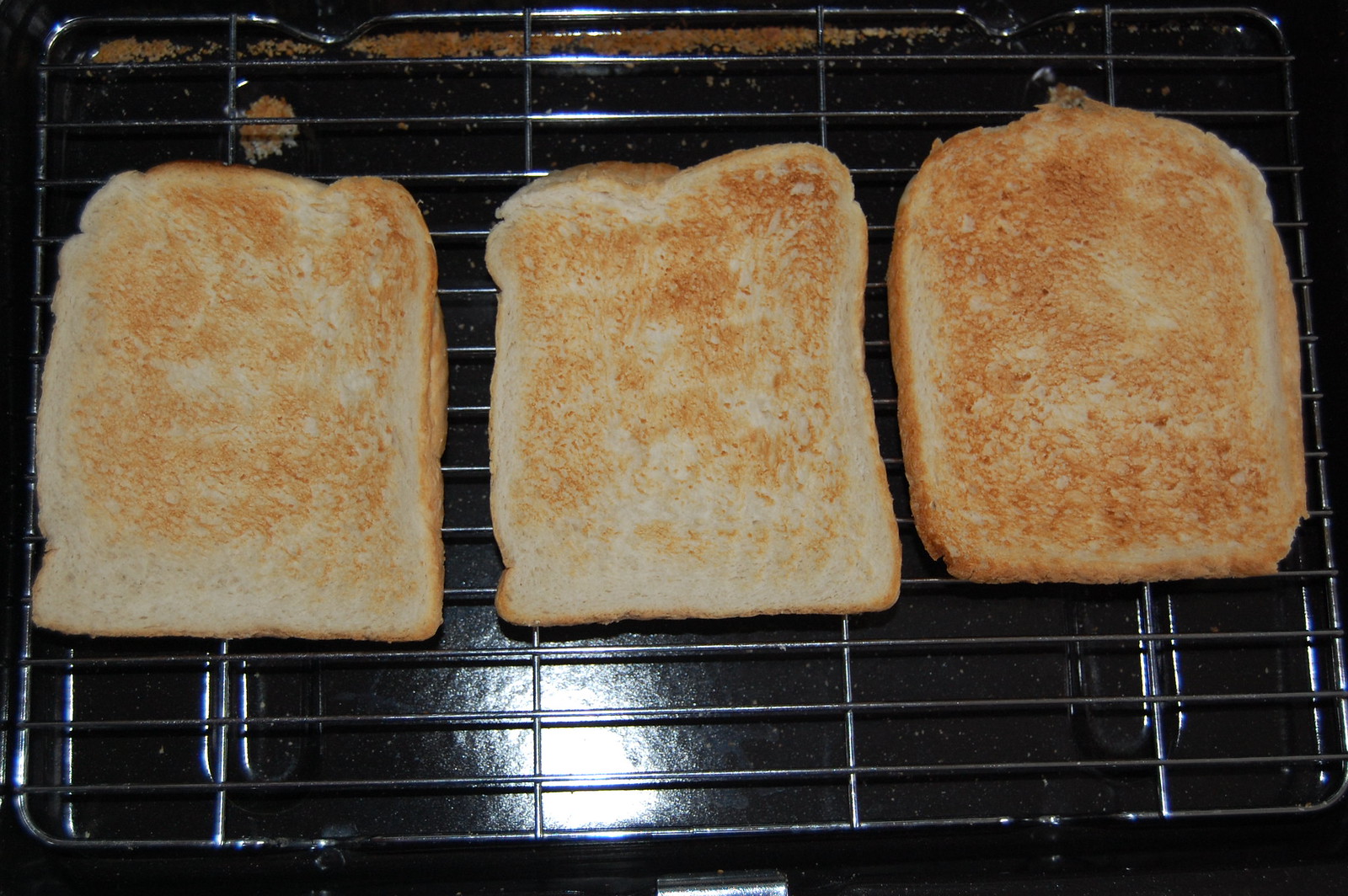This close-up horizontal color photograph captures three lightly toasted slices of white bread side-by-side, placed on a silver wire cooling rack. The wire rack sits atop a black speckled pan, which appears to be a standard 13 by 9 baking pan. The slices vary slightly in shade, with the two on the left being lighter and the one on the right slightly darker with a golden hue. The slice on the right is also the heel or end piece, identifiable by its rounder shape and thicker crust. There is a bright ball of light reflecting on the dark pan from above, creating a notable glare. The pan has a few breadcrumbs scattered along its top edge, with one larger crumb having fallen through the rack. The background is mostly obscured, but a small metal bracket at the bottom suggests the pan might be atop a countertop or stovetop.